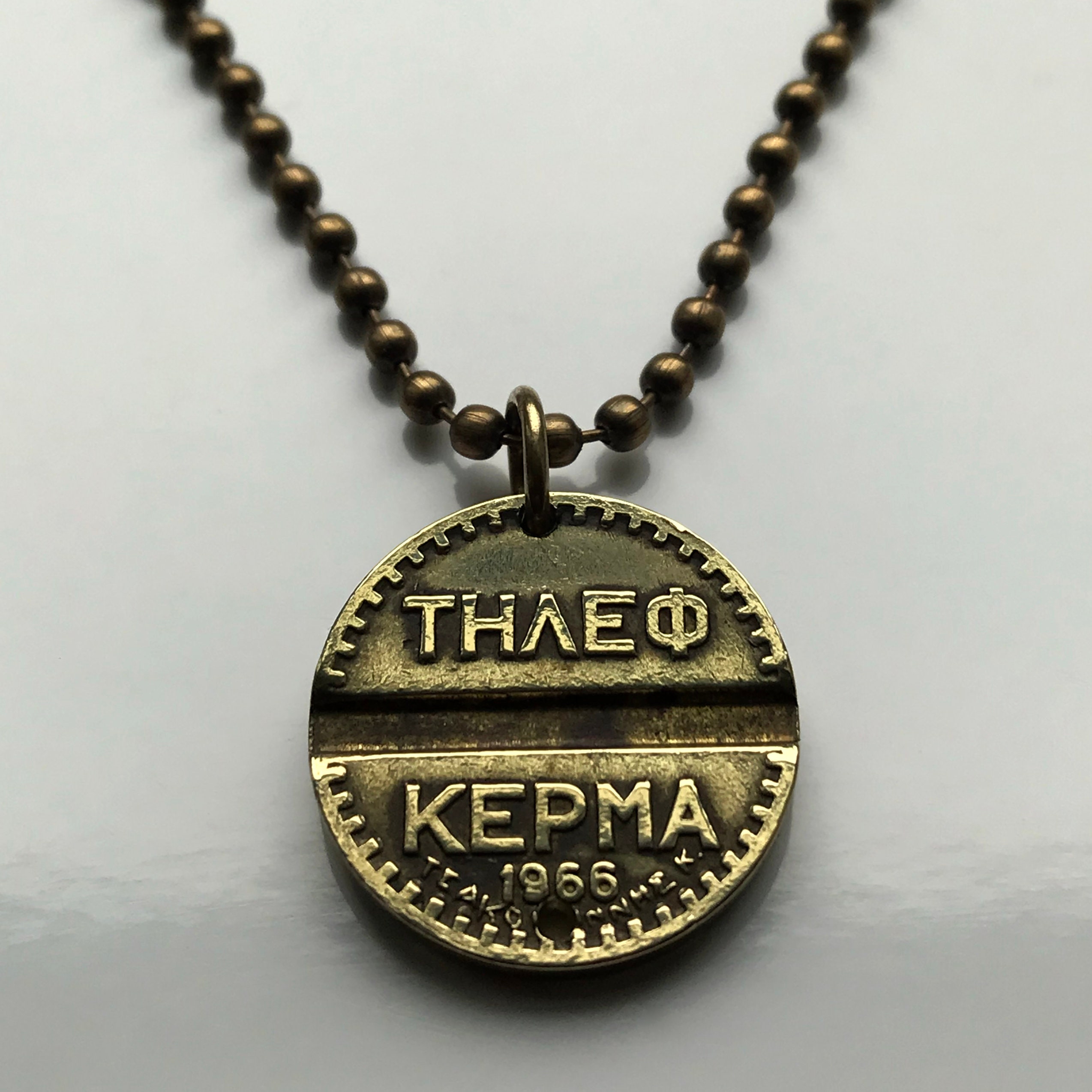The photograph features a close-up of a pendant or coin hanging from a ball chain necklace on a light gray background. The ball chain appears to be a dark bronzy, golden-brown color, typical of such chains. The pendant itself is circular, resembling a coin, with an edge that has little notches or pits around it. This coin-like pendant has seen some wear, evidenced by its faded golden hue and visible fingerprints. 

At the top of the pendant, the letters "T-H-A-E" are inscribed followed by an omega (Ω) symbol. Below this inscription, the word "K-E-P-M-A" is clearly engraved, and beneath it, the year "1966" is marked. Additionally, there is a horizontal ridge running across the middle of the pendant. The overall impression is that of a well-worn, darkened piece of jewelry, combining elements of both antiquity and personal use.